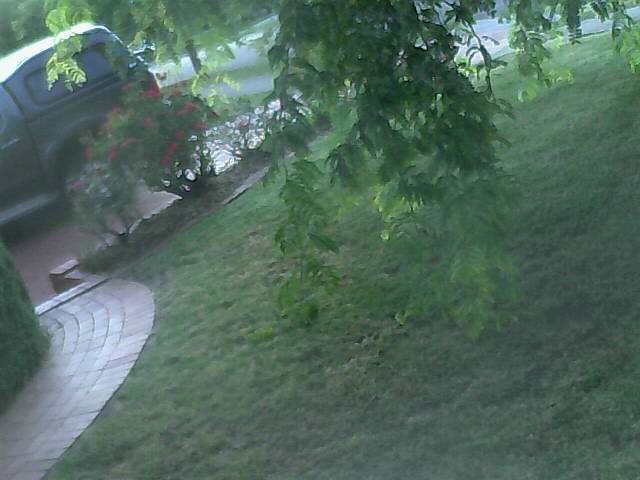A picturesque scene unfolds with a verdant, grassy hill rising prominently in the background. To the left, a pathway composed of carefully laid tiles winds its way through the landscape. Overhead, lush green leaves cascade gently, providing a natural canopy. In the foreground, a vibrant plant adorned with green leaves and colorful flowers adds a touch of natural beauty. A vehicle, either a truck or a car, can be seen driving away to the left, heading towards an area that looks like a black hole leading into a gray stream. The scene is rounded out by a sidewalk, which could possibly serve as a driveway, descending gracefully into the picturesque setting.